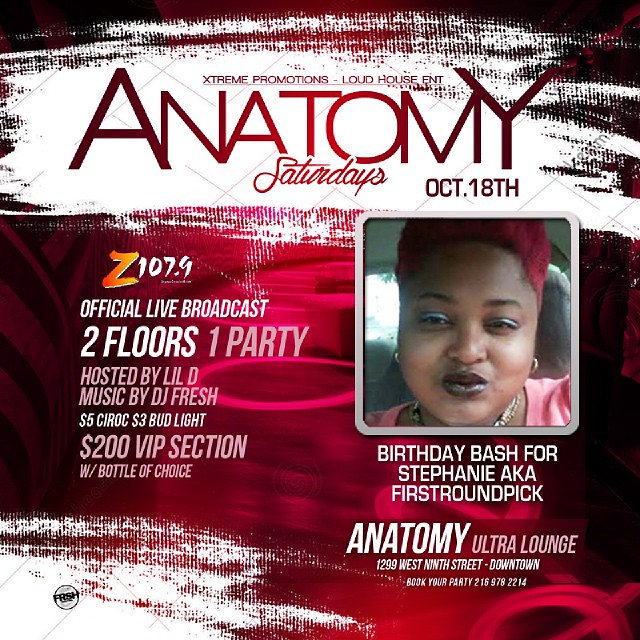This electronic flyer is predominantly in red, pink, and white, and advertises a club event by Extreme Promotions and Loud House Entertainment titled "Anatomy Saturdays" on October 18th. The centerpiece is the large "Anatomy" text in red with "Saturdays" in cursive below. To the right, beneath the letters "M" and "Y" of "Anatomy," the date "October 18th" is prominently displayed. 

A pink, decorative background with swirls and designs enhances the lower section of the flyer, where the radio station Z107.9 is highlighted, with the "Z" in orange and "107.9" in white. Following this, the flyer announces an official live broadcast featuring "Two Floors, One Party," hosted by Lil D with music by DJ Fresh. Drink specials include $5 CIROC and $3 Bud Light, and there's a VIP section available for $200 including a bottle of choice.

To the right side of the flyer, there is a square photograph of a woman with pink hair, blue eyeshadow, blackish-brown lipstick, and wearing ring earrings and a necklace, dressed in a peach outfit with only her shoulders visible. Below her photo, it states "Birthday Bash for Stephanie aka First Round Pick."

The information section at the bottom right corner provides the venue details: Anatomy Ultra Lounge at 1299 9th Street, Downtown. There is a call to action to "Book your party" with a phone number: 216-978-2214.